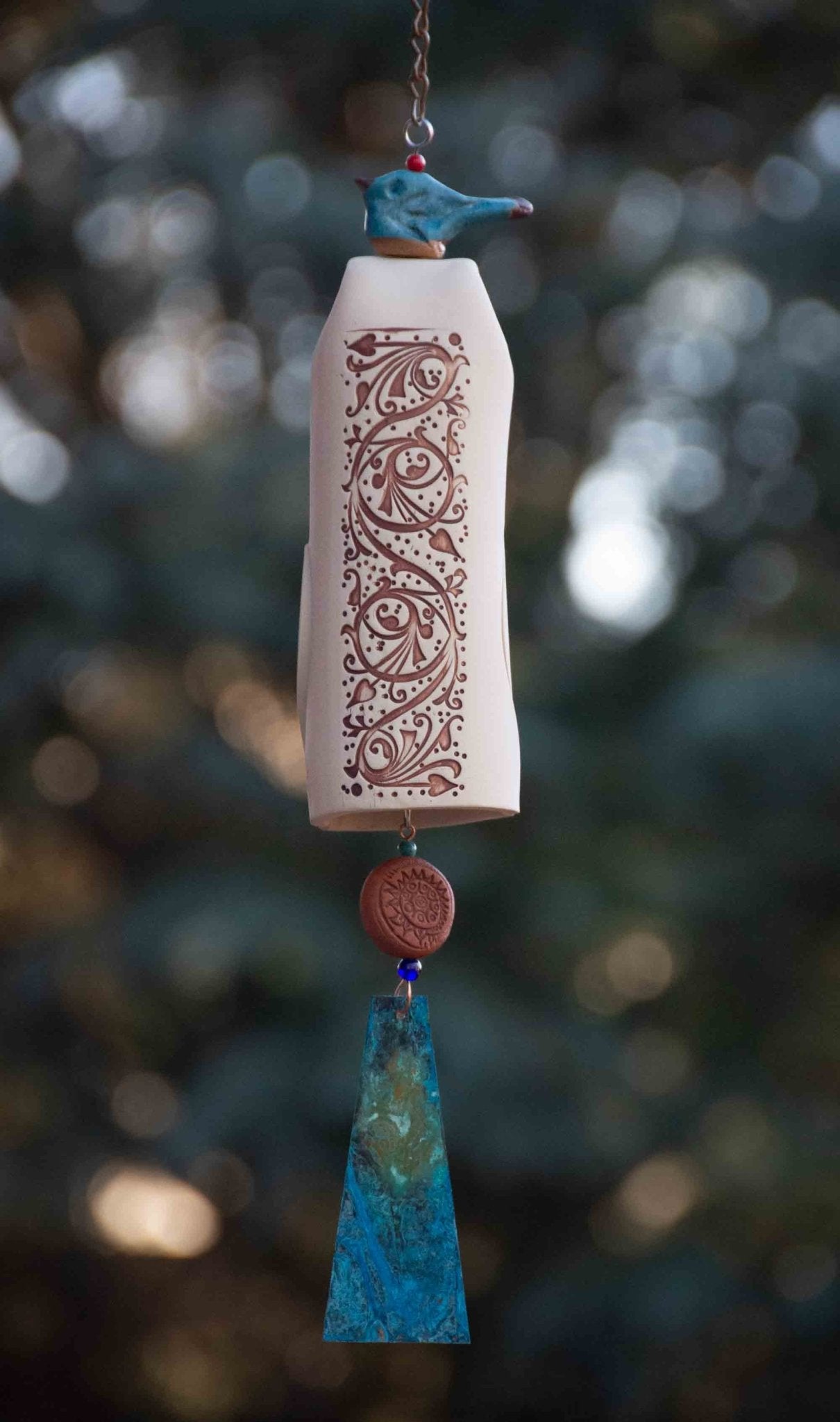The image depicts a wind chime hanging outside, accented by a background with a strong bokeh effect in tones of gray and green. The chime is suspended by a metal chain whose top part is not visible. At the top of the chime hangs a tiny blue clay figure resembling a bird. Beneath this bird is a vertically oriented, hollow, bone-white tube adorned with intricate, curvy brown designs that resemble leaves. Below the tube, another chain leads to a red clay-colored ball, followed by a flat, deep blue triangular piece that may have a glass or metallic texture.